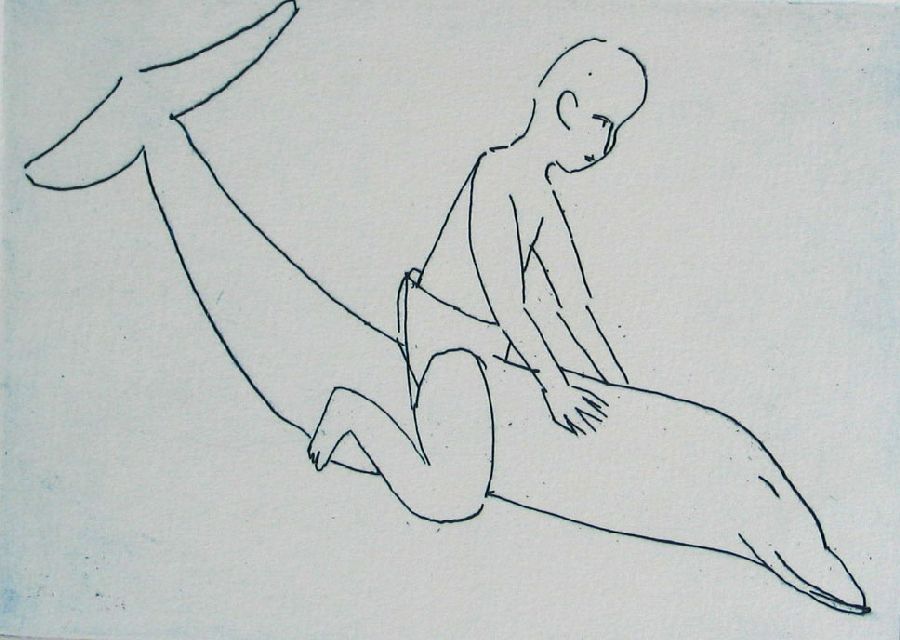The image is a very simple, black-and-white sketch of a boy riding what appears to be a dolphin. The drawing, which almost seems to be made from a single continuous line, exhibits a charmingly crude and intentionally simplistic style. The boy, who could be interpreted as wearing either an oversized swimsuit or a diaper, is depicted with hands and feet that seem to be hugging the dolphin’s body—one hand is visible while the other wraps around the back, and his legs are positioned as if he’s riding the dolphin like a pony. The dolphin, which is missing several key features such as side fins and a dorsal fin, is drawn with its closed eye and a slight smile, giving it a content appearance. There are noticeable gaps in the lines that form the boy and the dolphin, such as around the ears, the dolphin's tail, and where the boy's legs meet the dolphin's back. Despite these gaps, the image clearly conveys the joyous scene of the boy and the dolphin, with the dolphin swimming from the upper left corner to the lower right. The overall impression is one of innocence and happiness, making it easily identifiable despite its simplistic execution.